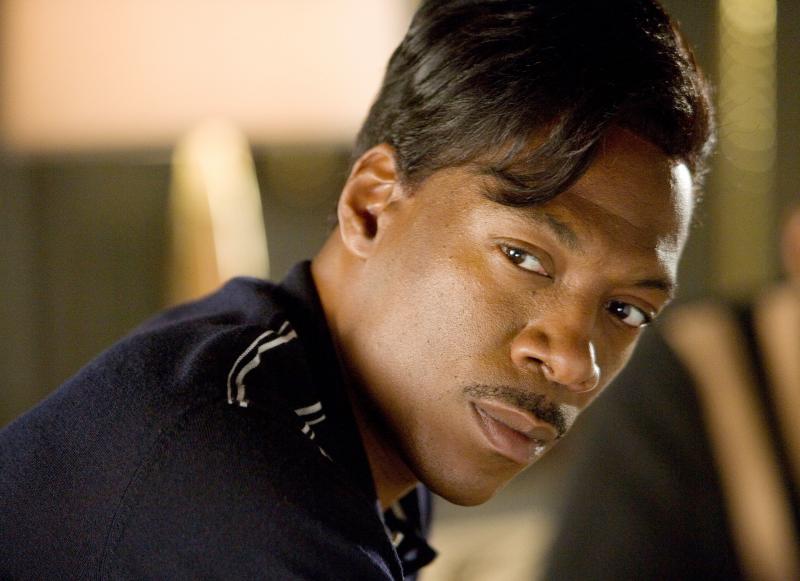The photograph captures a close-up side profile of an African American gentleman, reminiscent of Eddie Murphy. He appears to be in his early thirties and is slightly tilted to the right, gazing towards the viewer. His neatly coiffed black hair is parted on the left, with a few strands falling onto his forehead. He sports a distinct black mustache. The man is dressed in a dark blue shirt adorned with thin white stripes near the shoulders. The background is blurred, with hints of green and cream colors, possibly depicting a soft, out-of-focus setting with a white ceiling and a yellowish pillar. The image is rectangular in shape and possibly includes another figure in the background, though it remains indistinct.